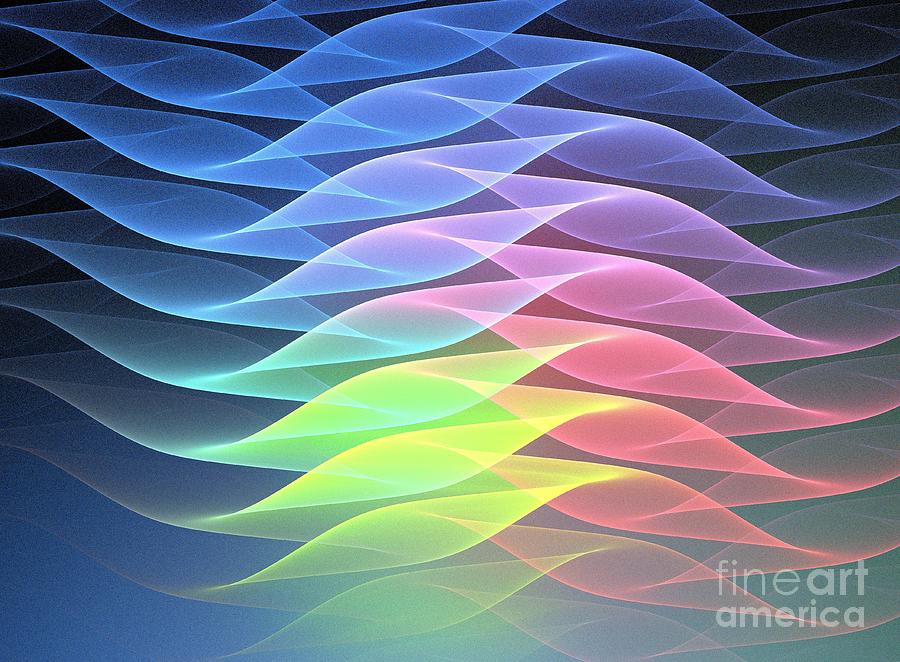This image features an expertly crafted, computer-generated wave pattern set against a gradient background that transitions from black at the top to blue towards the bottom. The waves, or ribbon-like structures, weave and fold over each other, creating a fluid and dynamic composition. These ribbon waves exhibit a rich array of colors: starting with various shades of blue near the top, then transitioning through purple, pink, red, yellow, and green, before finally settling into darker tones at the bottom. Each ribbon-like wave is distinct in color, lending a unique and vibrant quality to the scene. In the bottom right corner, the text "Fine Art America" is clearly visible, identifying the source of this intricate artwork. The overall effect is a mesmerizing blend of colors and shapes, meticulously arranged to captivate the viewer.